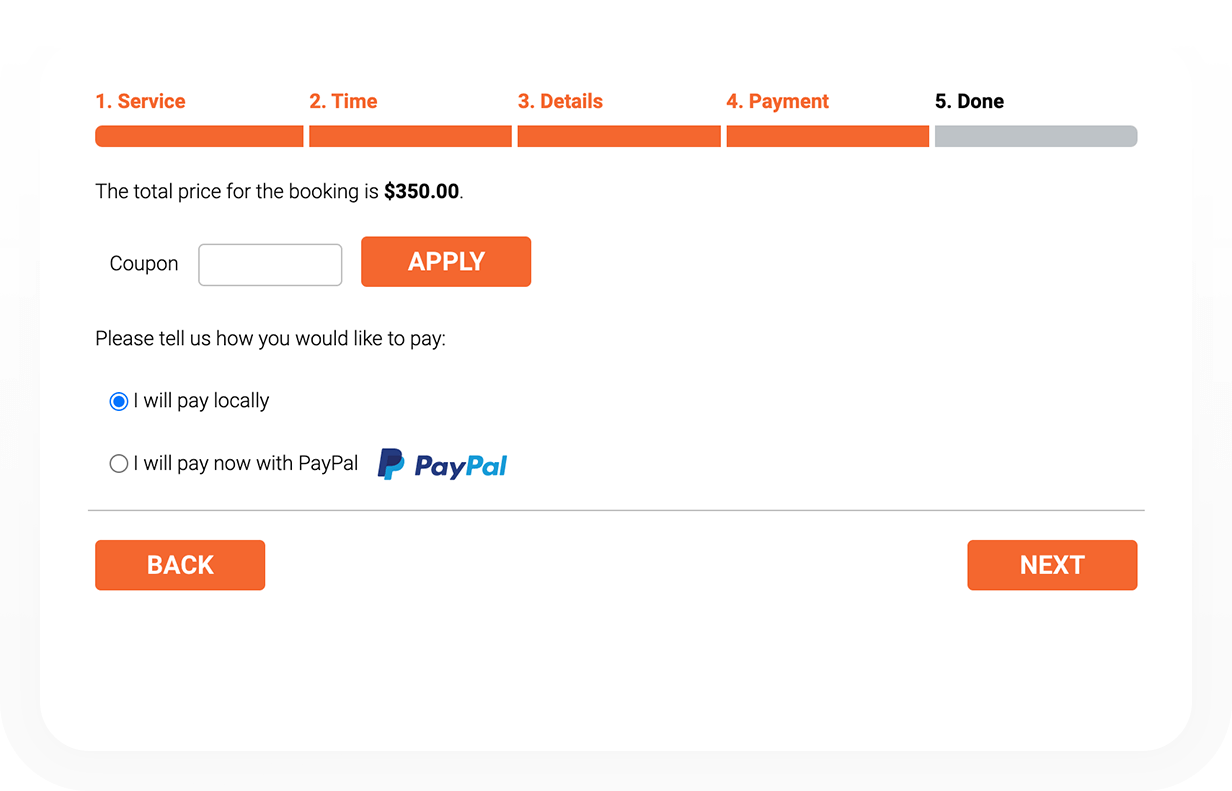The image depicts a detailed webpage dedicated to the process of booking a service, divided into five clearly defined steps: 

1. **Service**
2. **Time**
3. **Details**
4. **Payment**
5. **Done**

The initial four steps, labeled "Service," "Time," "Details," and "Payment," are highlighted in orange, signifying progress through the booking process. Below these steps, the webpage prominently displays the total booking price of **$350** in bold black text.

Further down, there is a section for applying a coupon, accompanied by an orange "Apply" button. Beneath this section, a prompt states, "Please tell us how you would like to pay," followed by two payment options in the form of boxes:

- **I will pay locally:** Marked with a blue check mark, this option indicates it is currently selected.
- **I will pay now with PayPal:** Alongside the PayPal logo, which features two shades of blue—the word 'Pay' in darker blue and 'Pal' in lighter blue.

Finally, at the bottom of the webpage, there are two additional orange buttons labeled "Back" and "Next," both featuring white text set against a predominantly white background, with the total due amount in bold text to draw attention.